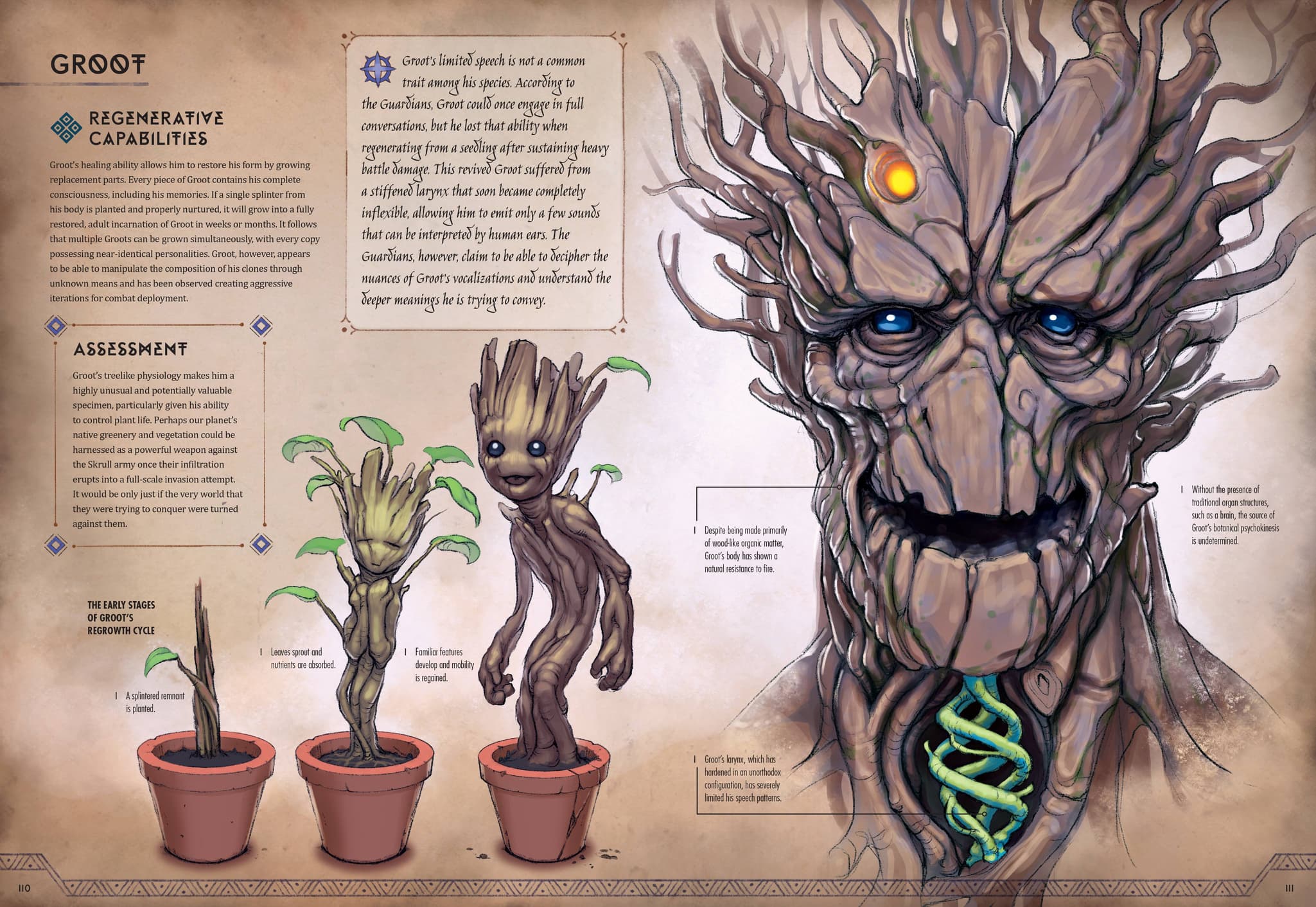The image is a detailed illustration of Groot, a character from Guardians of the Galaxy, presented as conceptual artwork. At the top left, the word "Groot" is prominently displayed, accompanied by a small, hard-to-read paragraph titled "Regenerative Capabilities." Below this, another small, somewhat illegible box labeled "Assessment" provides additional information.

To the right, a cursive text box adds further complexity, though its contents are difficult to discern due to the font and size. The illustration features a growth sequence of Groot, starting from the bottom left corner with three versions of Groot in flower pots. The first version shows him as a small stick, gradually sprouting leaves. In the next stage, Groot is slightly taller with more pronounced features. Finally, he is depicted as a mature, tree-like figure, characterized by gnarled branches extending from his head, vibrant blue eyes, an orange element near the top, and a green object around his neck.

The background of the entire artwork resembles textured parchment, adding an aged, natural feel to the piece.